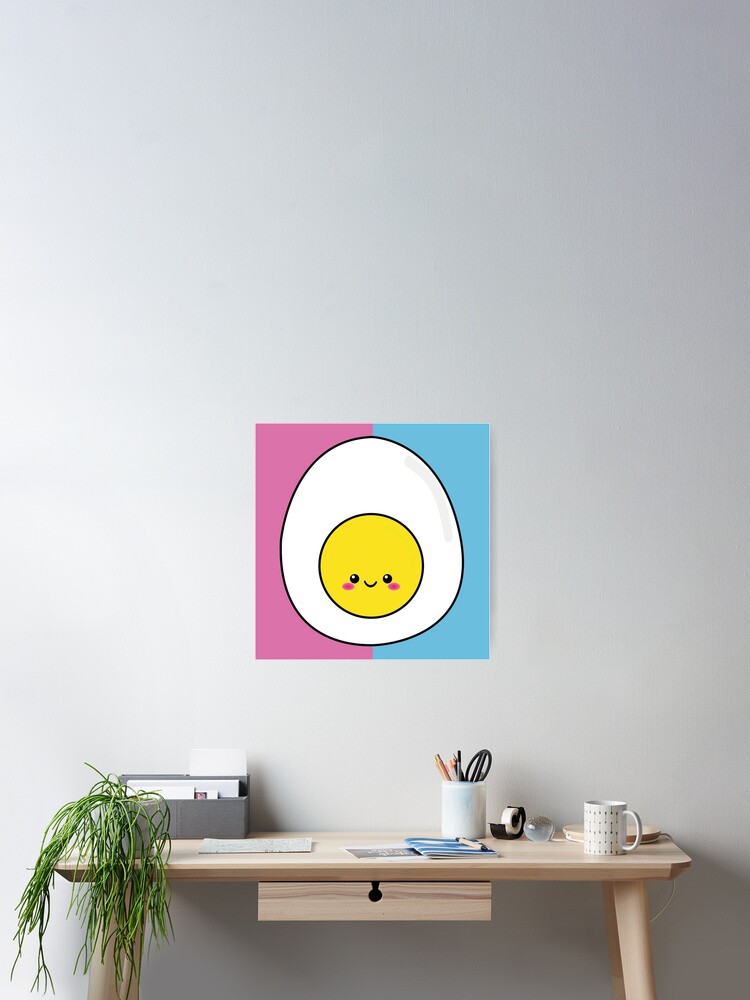The image depicts a bright indoor scene, likely taken during the daytime, featuring a minimalistic office setting with a white wall background. Central to the picture is a light wooden desk positioned against the wall. The desk is adorned with various items, including a green plant in a grey container on the left-hand side, its leaves trailing off the desk. On the right side, there is a white table lamp and a white coffee mug decorated with a linear grey design. Scattered across the desk are papers, a tape dispenser, a paper weight, and a white, marble-like pencil holder containing scissors and various writing utensils. There is also a gray receptacle for holding papers.

Above the desk hangs a two-toned painting with the left side pink and the right side blue. The artwork features a cartooned image of a sliced hard-boiled egg, with a yellow yolk in the center that has eyes, a mouth, and blushed cheeks, giving it a smiling expression. The desk appears to have a drawer in the center beneath the tabletop. The absence of a chair suggests the photographer may have stepped back to capture the image.